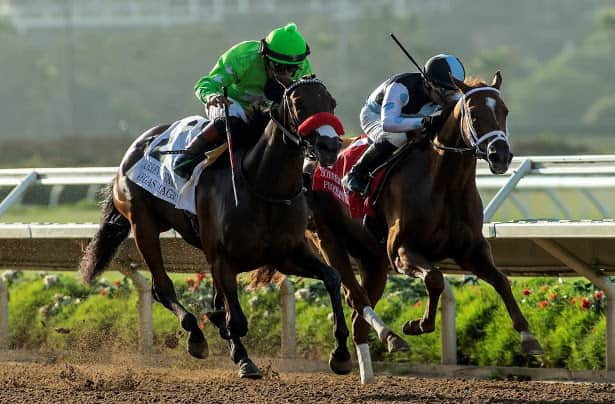This is a detailed photographic image of two dark horses racing on a brown dirt racetrack outdoors during the day. In the foreground, a horse with a red noseband races prominently. Its jockey is dressed in a green outfit, wears a green hat with a black headband, and has a blanket under the saddle that appears to have the letters "G-A-S-L-A" on it. The horse trailing behind wears a white bridle, and its jockey is attired in a black and white jersey, with a black and blue helmet. Both jockeys wear black boots. The horses appear to be moving at high speed, kicking up dirt as they go. Surrounding the track, the background features a metal fence with bushes adorned with red flowers, and beyond that, some faded, out-of-focus gray trees. This scene is set against a subtly visible outline of a distant mountain, completing the vibrant and dynamic depiction of an intense race.